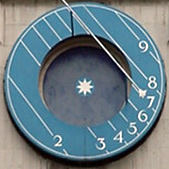This small square photograph features a distinctive round, flat blue ring, possibly crafted from wood. The ring is perfectly circular with an equally circular cutout at its center. It rests on a smooth, gray surface. Inside the cutout, a dark gray circle bears an elegantly painted white star featuring eight points. Adjacent to the edges of this circle are diagonal lines, running from the upper left to the lower right, numbered sequentially from 2 to 9 along the bottom and right borders. An additional thin vertical dark line is visible in the upper left quadrant of the circle. Although the arrangement and markings suggest it may be a form of a sundial, there are no labels or indicators confirming its exact purpose.